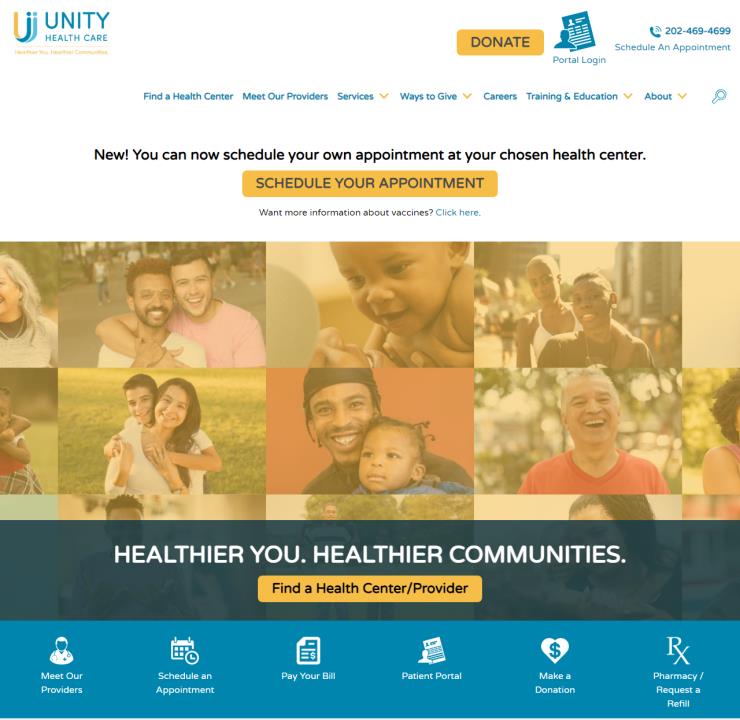The image depicts a detailed web page layout for Unity Healthcare, featuring various sections and information prominently displayed. The upper portion of the page has a white background on the left side, with the text "Unity Healthcare" written in a teal color. Below this, there are additional words that are blurry and hard to read due to the yellow background.

On the right side, there is a yellow rectangle with the word "DONATE" written in all caps in black text. Below it, in the same teal color, the phrases "Portal Login" and "Schedule an Appointment" are written alongside an icon of a phone and the contact number 202-469-4699, which suggests the location is in Washington, DC.

Beneath these elements, there are a series of teal tabs with white text that says:
- "Find a Center"
- "Meet Our Providers"
- "Services" (with a yellow arrow pointing down)
- "Ways to Give" (with a yellow arrow pointing down)
- "Careers"
- "Training"
- "Education" (with a yellow arrow pointing down)
- "About" (with a yellow arrow pointing down)

To the right of these tabs, there's an icon that appears to be a magnifying glass, indicating a search function.

Further down the page, in black text, it reads, "New! You can now schedule your own appointment at your chosen health center." Following this announcement, there's an orange rectangle with black text that says, "Schedule Your Appointment."

Below this section, it asks users if they want more information about vaccines, ending with "Go to?" followed by blue text that says "Click Here."

The page also features a collage of images showing diverse individuals who might visit Unity Healthcare, including babies, a baby with a father, an older man, and various couples.

Towards the bottom, against a blue background, there is white text proclaiming, "Healthier You, Healthier Communities." Lastly, another orange rectangle box with text in black and blue says, "Find a Health Center / Provider."

This comprehensive layout is designed to provide quick and easy access to essential healthcare services and information.